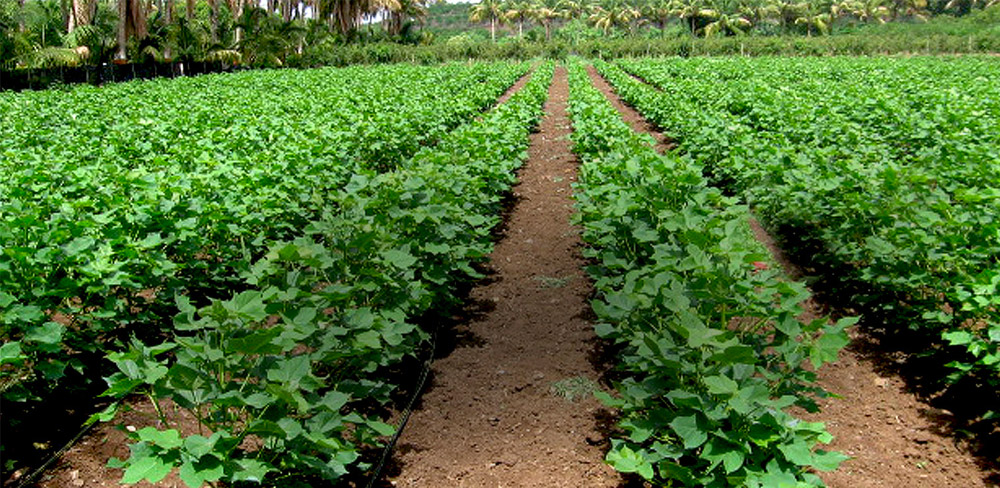The image depicts an expansive farm scene with numerous rows of lush, green plants that are believed to be sweet potato plants, characterized by their large leaves. These plants are low to the ground, and the soil between them appears brown and muddy. Prominent dirt paths run between the rows, guiding the eye towards the back of the farm. Along these paths, there are hoses or wires laid out, perhaps for irrigation. In the distant background, a line of palm trees stands tall, flanked by a green, terraced hillside that adds depth to the scene. The left-hand side of the image similarly features palm trees stretching off into the distance. The serene setting, free of any text, provides a vivid snapshot of agricultural life, from the rich earth to the encompassing greenery.